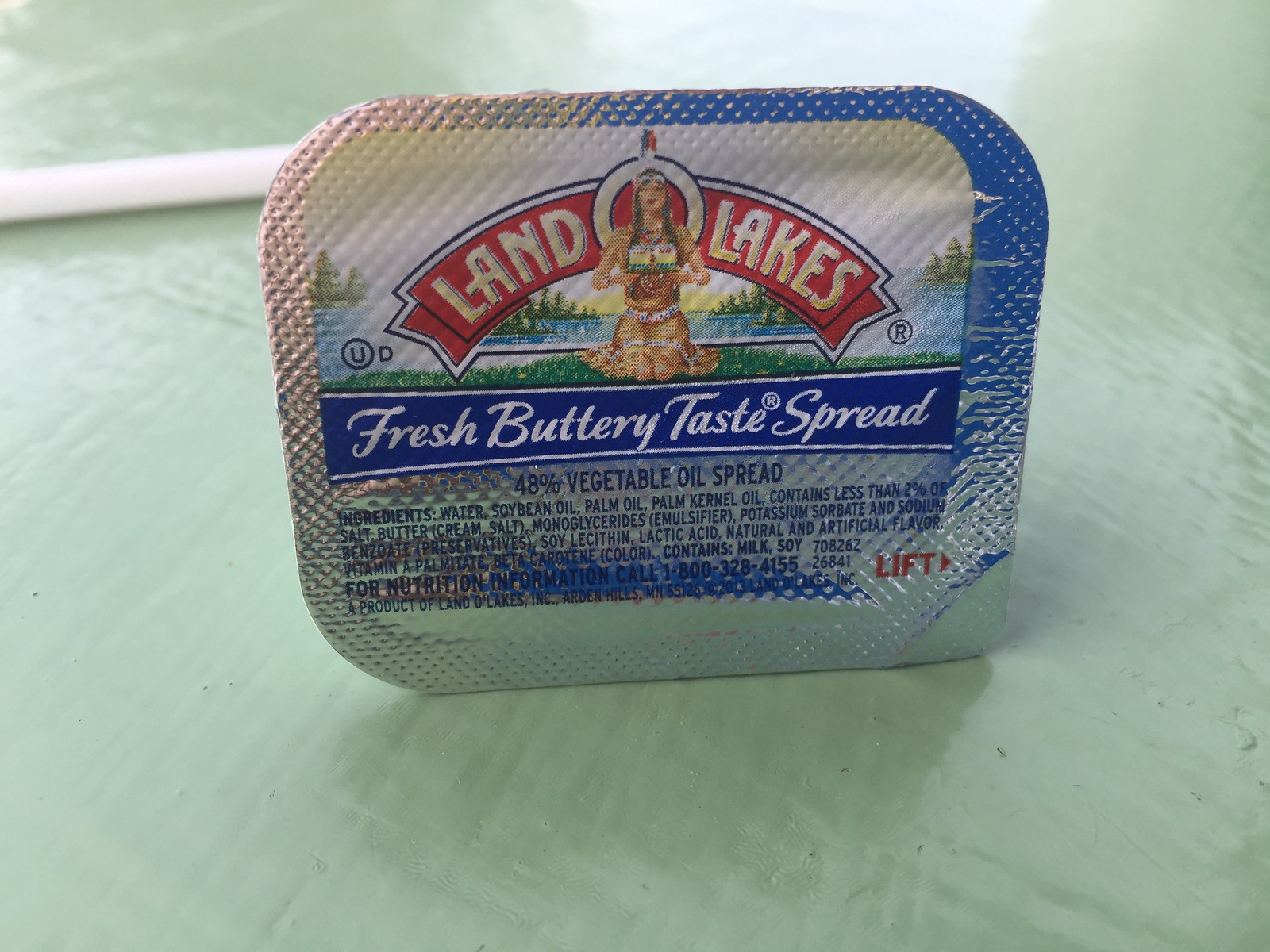This photograph captures a small, individually-sized container of Land O' Lakes butter, typically distributed at restaurants. The container is sealed with a metallic foil lid, prominently featuring the brand's iconic logo. A red ribbon-like banner stretches across the foil, emblazoned with the words "Land O' Lakes" in white. 

Below the brand name, the logo depicts a Native American woman in traditional buckskin attire, holding a plate of butter. She is adorned with a feather in her hair, reinforcing a culturally inspired design. Beneath this image, the phrase "Fresh Buttery Taste Spread" is elegantly written in white cursive on a blue backdrop.

The product details continue with a clarification that this spread contains "48% Olive Oil." Further down, a list of ingredients is visible, printed in dark blue text. Situated on the right side of the container, the red word "Lift" accompanied by a small triangular arrow indicates where to peel back the foil to access the butter.

The foil-sealed butter rests on a shiny, textured green countertop, which adds a vibrant contrast to the container's metallic sheen.